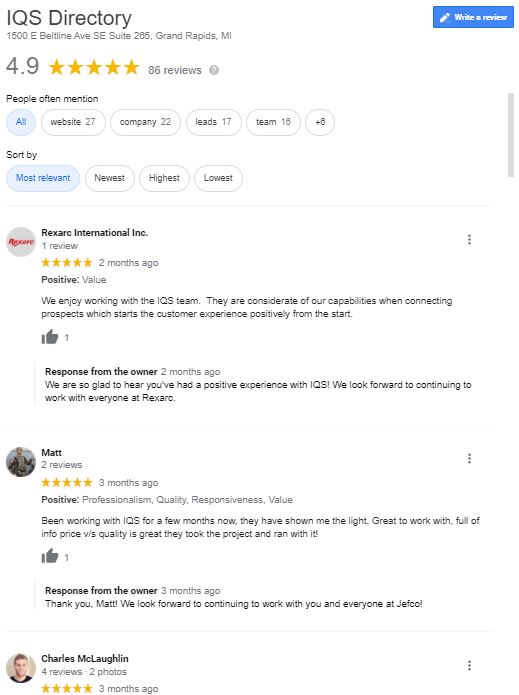Screenshot of an IQS Directory Review Page

The image is a screenshot of a computer monitor displaying an IQS Directory review page. At the top of the screen, the IQS Directory logo is prominently visible. On the right-hand side, there's a blue button labeled "Write Review." Below the button is some text, too small to read clearly without enlargement.

The address listed on the screen reads: "1500 E Belton of SE, Suite 285, Grand Rapids, MI." The IQS Directory has an impressive rating of 4.9 stars based on 86 reviews. Frequently mentioned keywords in the reviews include "Website" (27 mentions), "Company" (22 mentions), "Lead" (17 mentions), and "Team" (16 mentions), with an additional 6 unspecified terms.

A sorting option for the reviews is highlighted, indicating that the reviews are currently sorted by "Most Relevant." Other sorting options include "Newest," "Highest," and "Lowest," each encased in small rectangles for selection.

The first visible review is by Resan International Inc., posted two months ago, with a five-star rating. The reviewer appreciates the positive value and mentions enjoying the collaboration with the IQS team, noting their consideration of capabilities when connecting prospects. This particular review has garnered one like. The company's response two months ago expresses gratitude and eagerness to continue the collaborative relationship with IQS.

Following that, Matt, who has two reviews and a faint picture of himself attached (though blurry), posted a review three months ago. He also gave a five-star rating, commending the professionalism, quality, responsiveness, and value he experienced while working with IQS. He praised the team for showing him "the light" and successfully handling the project, balancing price and quality. This review also has one like. IQS responded three months ago, thanking Matt and expressing anticipation for future collaborations with JetPro.

At the bottom of the screenshot, another review is faintly seen from Charlie McLaughlin, who has four reviews and a partial, out-of-focus profile image. However, the content of Charlie's review is not legible in the image.